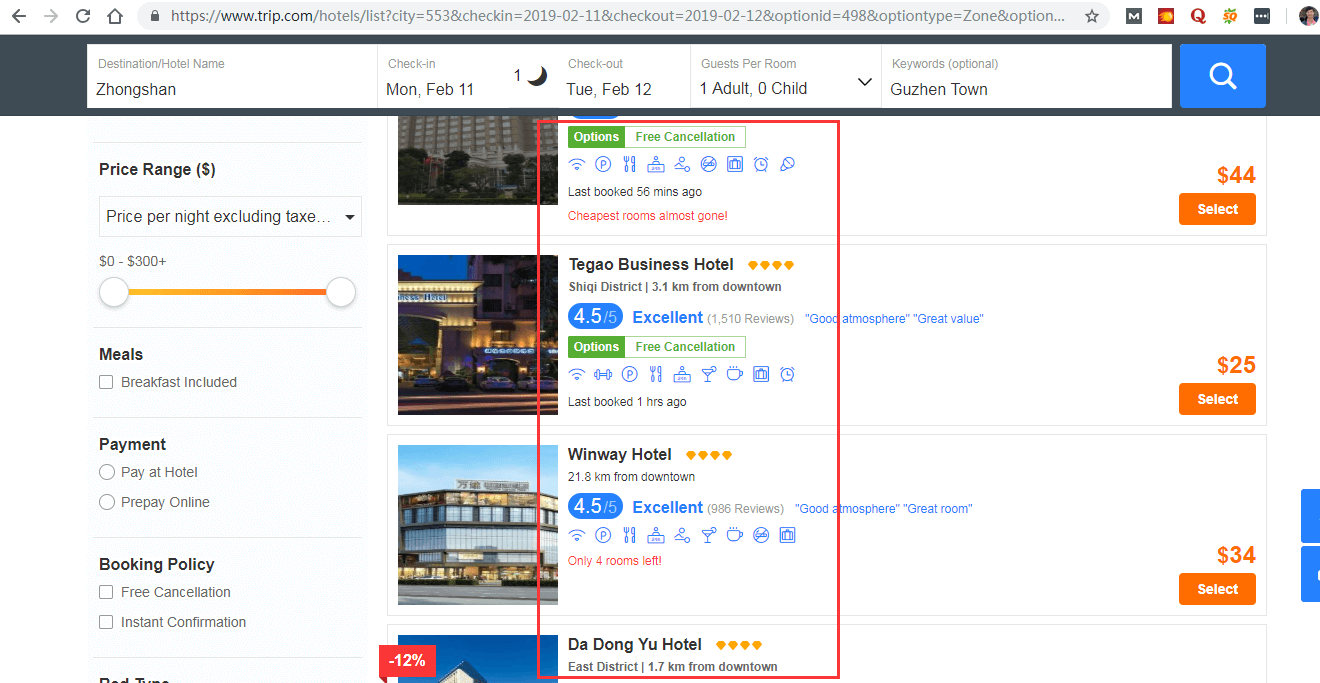The rectangular image, oriented with the long side running horizontally, depicts a webpage from trip.com where a user is searching for a hotel. At the top of the page, there is a search bar section outlined in black. It displays the following details: the destination is Zhongshan, the check-in date is Monday, February 11th, and the check-out date is Tuesday, February 12th. The reservation is for one adult with no children, and the keywords entered are "Gusen Town." There is a blue search button with a search icon located on the far right of this section.

Beneath the search bar, on the left side, there is a column listing filtering options which include price range, meals, payment methods, and booking policies. The current price range is set to $0 to $300. Under the meals section, the "breakfast included" option is noted. The payment section offers choices of "pay at hotel" or "prepay online." The booking policy section highlights "free cancellation" and "instant confirmation."

In the main content area towards the middle of the page, there are details of four hotels listed, with three specifically named: Checkout Business Hotel, Winway Hotel, and Dongyu Hotel, each accompanied by their respective prices.